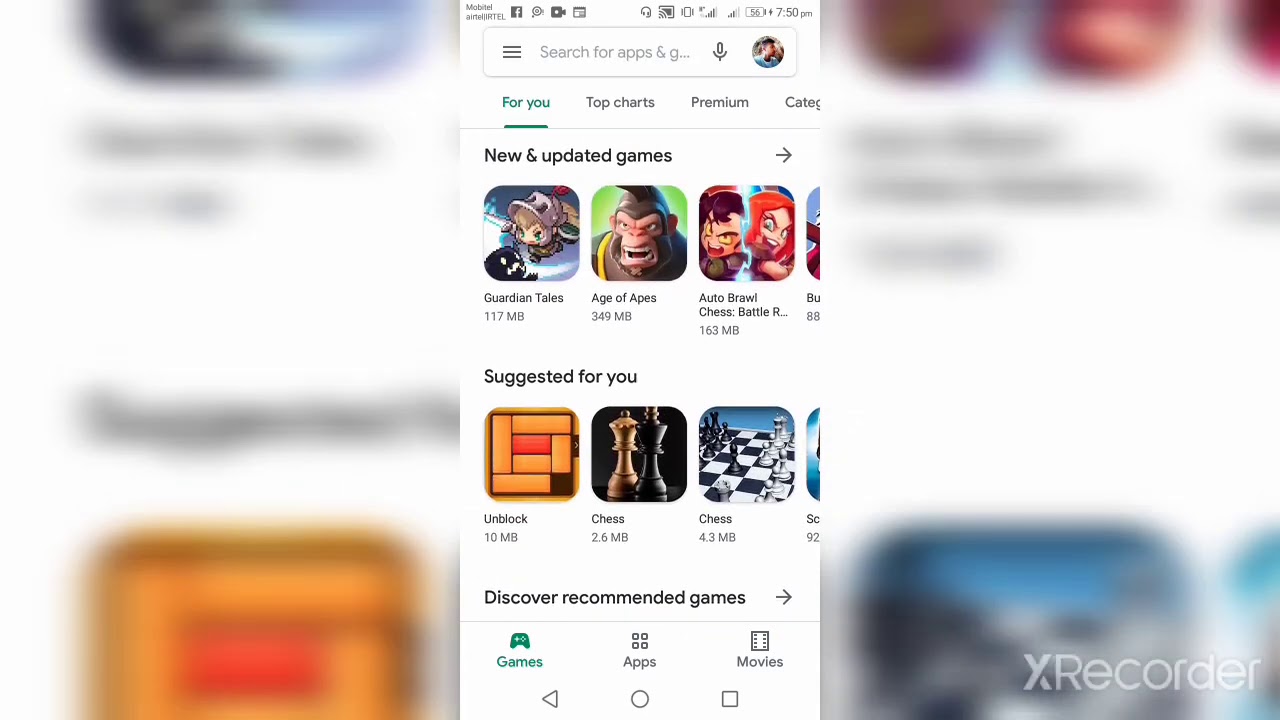This image depicts a mobile interface of what appears to be an app store. The layout is divided into two primary sections, centered by a vertical column. The view appears to be from a smartphone, showcased in a vertical orientation.

At the very top of the image, there's a cluster of icons, including a discernible question mark, though the rest are too small to identify properly. Below the icons, there is a search field with a partial phrase "search for apps," followed by a truncated "G..." ending with ellipses. The search field includes a microphone icon for voice search and a small circular icon resembling a user profile picture.

Underneath this, there are several navigational tabs: "For you" is currently selected, and next to it are "Top charts," "Premium," and a partially cut-off "Categories."

Directly below these tabs, a section labeled "New and updated games" displays various game options, complete with icons and the sizes of each game. One of the listed games is "Age of Apes." 

Further down the interface, the section "Suggested for you" presents more app recommendations, primarily games. Below that, another section titled "Discover recommended games" offers additional suggestions for games, apps, and movies.

The background of the image is slightly grayed out with additional icons from the app store, which are notably larger and also mostly illegible, adding a depth effect to the overall layout.